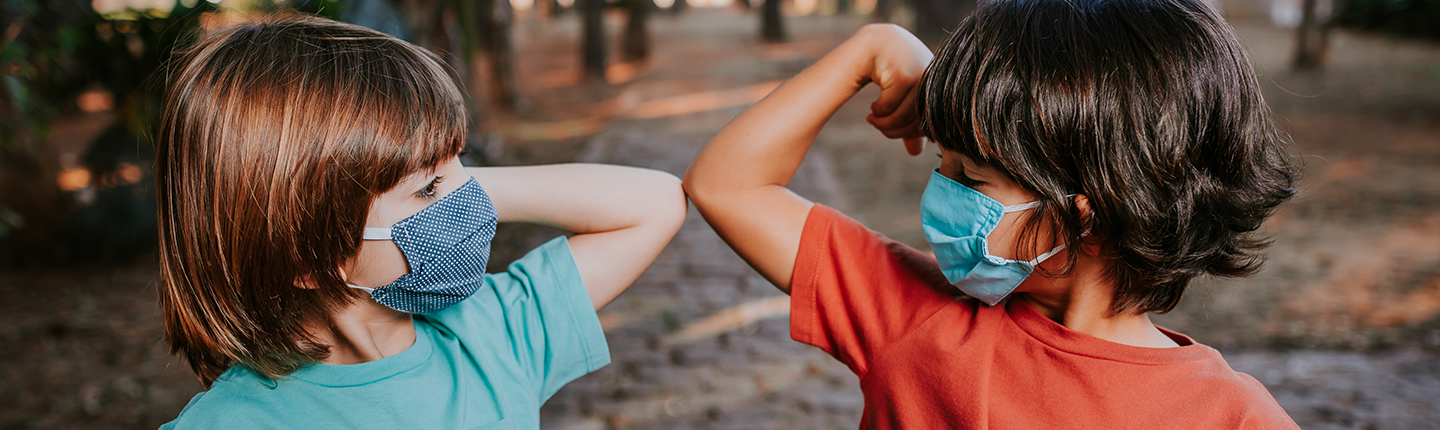This detailed photograph, horizontally oriented, captures a realistic scene featuring two young boys on what appears to be a cobblestone street, likely outdoors though the setting remains somewhat ambiguous. The main focus is on the boys, who are approximately 5-7 years old, engaging in a COVID-era greeting by bumping elbows while striking a muscle-flex pose.

On the left, a boy with fair skin and chestnut brown hair that reaches his shoulders wears an aquamarine short-sleeved T-shirt. His face is partially covered by a dark blue cloth mask adorned with white polka dots and white straps. Opposite him, the boy on the right has a slightly darker complexion and black hair of similar shoulder-length. He sports a red-orange short-sleeved T-shirt and a blue surgical-style mask with white straps.

Both boys are turned towards each other, making eye contact while their right and left elbows meet. Behind them, the slightly blurred background hints at a stone pathway or cobblestone street, but the specific details remain indistinct, keeping the focal point firmly on the boys and their playful yet socially conscious interaction.